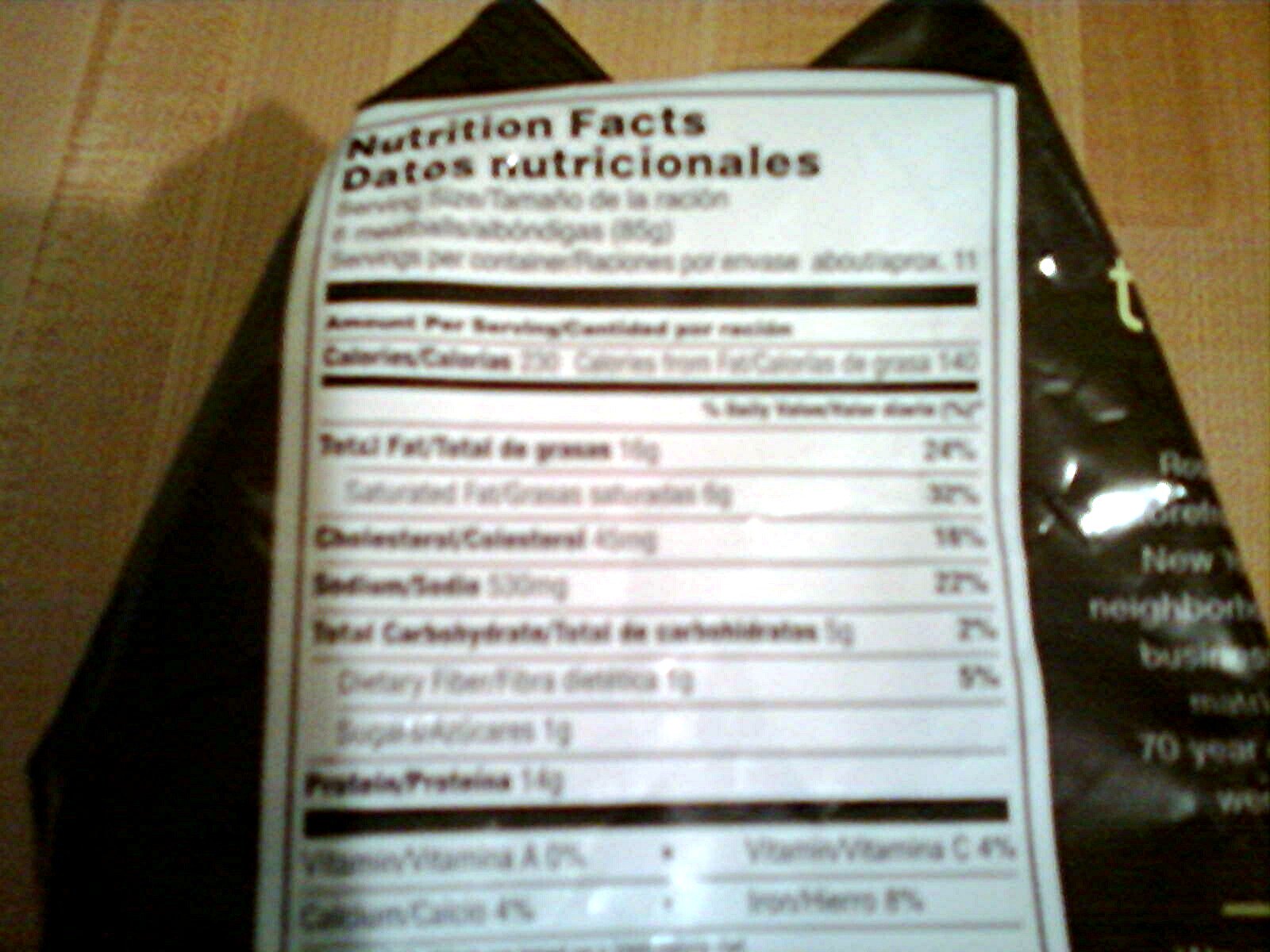The image is a color photograph depicting a nutritional facts label on a package of dates. The photograph appears to be of poor quality, resulting in a blurry and grainy image with misrepresented colors. The label is set against a black packet with a light brown, vertically paneled wooden floor in the background. There are unintended specks of green, black, and pink visible in the image.

Despite the blurriness, some details on the white label with black text can be discerned. At the top, the label reads "Nutrition Facts" followed by "Datos Nutricionales" in Spanish. It lists nutritional information with both English and Spanish translations, such as serving size (seis meatballs, albóndigas), and servings per container (raciones por envase), though the text is mostly illegible.

The label includes categories like total fat (16g, 24% daily value), saturated fat (32%), cholesterol (16%), sodium (530mg, 22%), total carbohydrates, dietary fiber (5%), protein (14g), calcium (4%), iron (8%), and vitamin C (4%). Percent daily values and specific measurements are indistinct but hint at a highly detailed breakdown of the nutritional content of the dates.